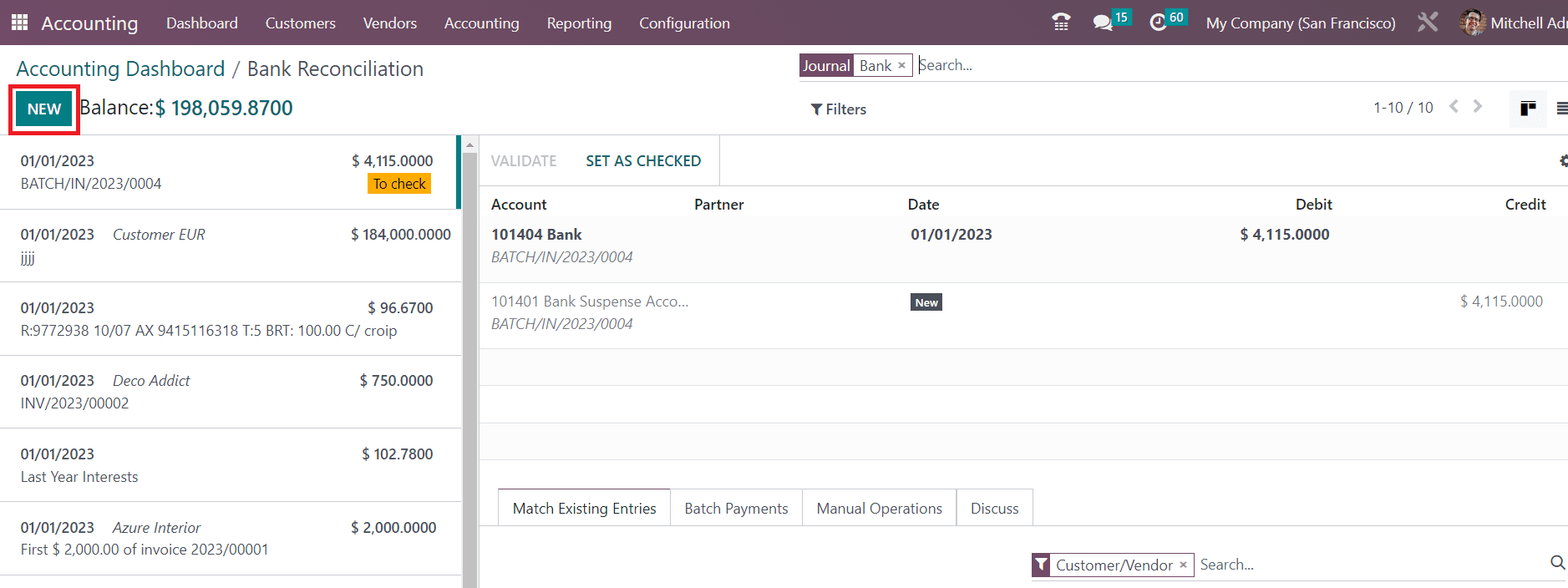The image displays a web application interface dedicated to financial management. At the top, a purple navigation bar lists several sections: "Accounting," "Dashboard," "Customers," "Vendors," "Accounting" (repeated), "Reporting," and "Configuration." On the right side of this bar, it displays "My Company, San Francisco," followed by "Mitchell," though the last name is obscured.

Beneath the navigation bar, a secondary blue bar features options such as "Accounting," "Dashboard," and "Bank Reconciliation." Highlighted in this section is a teal button labeled "New," which is outlined in red. 

The main content area includes various financial details. Notably, there is an account balance of $198,059.87. Additional information includes "Batch 1123" with a transaction amount of $4,115,000 and a check identified as "1123" with a value of $184 million. Further, account "101-404 Bank 4" shows an amount of $1,115,000 and a reference to last year's interest marked as "102."